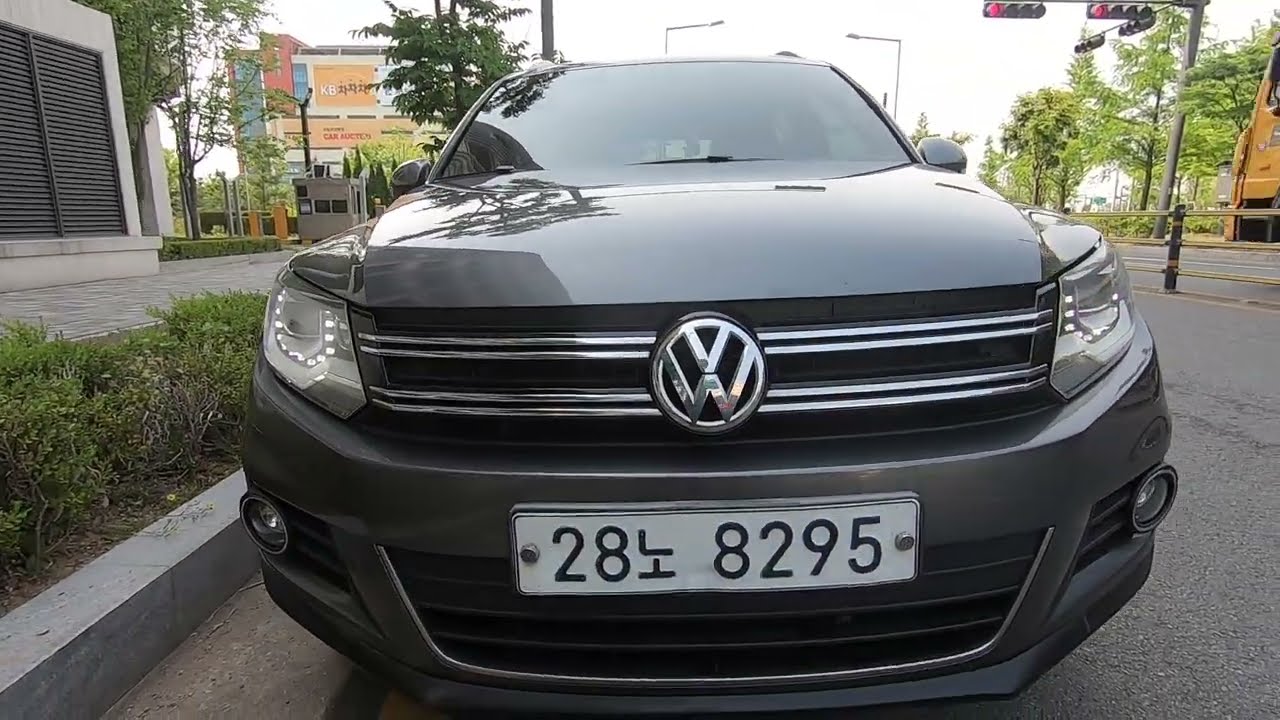In this detailed photograph, we see the front end and grille of a dark gray Volkswagen vehicle, prominently featuring the chrome VW emblem in the center. The license plate reads 288295 in black lettering on a white background. The car is parked on a street adjacent to a gray pavement sidewalk, with short green shrubs lining its edge. On the left side of the image, there is a gray metal wall with louvers, likely housing equipment such as air conditioning units. A variety of urban elements are visible: trees, multi-story buildings with a mix of English and Japanese signage, and streetlights indicating red. A multi-lane roadway and a yellow train can be seen on the right, adding to the bustling urban environment. Additionally, the front end of a truck is just entering the frame from the left. The overall setting appears to be in Japan, captured on a bright day with a light-colored sky.